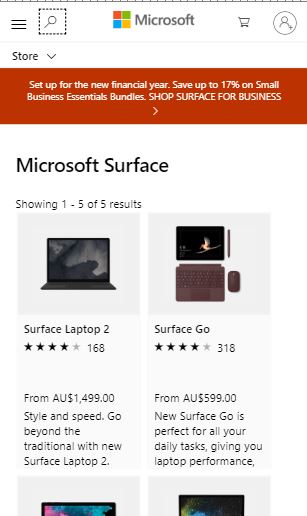This detailed caption describes the main page of the Microsoft Store and its layout:

---

The image captures the main interface of the Microsoft Store, with a clean and organized design. On the upper left-hand side, there is a context menu indicated by three horizontal lines. Next to it is a search button represented by a magnifying glass icon encased in a square. The iconic Microsoft logo, composed of four colored squares (red, green, blue, and yellow), is prominently displayed at the top. Adjacent to the logo are a cart icon resembling a grocery cart and a profile icon illustrated as a humanoid figure within a circle.

A red banner near the top announces the ability to "Set up a new financial year" and offers "up to 70% off on small business essential bundles." Below this, another promotional message urges customers to "Shop Surface for Business."

The main content area has a white background with black lettering. It showcases Microsoft's Surface lineup, highlighting that 5 of 5 results are being displayed. Featured prominently are:

- **Microsoft Surface Laptop 2:** Rated four stars based on 168 reviews. Priced at AUD $1,499, it's described with the tagline "Style and Speed, Go Beyond Traditional" to emphasize its capabilities.
- **Surface Go:** Also rated four stars, but with 318 reviews. It starts at AUD $599 and is touted as "perfect for all your daily tasks, giving you laptop performance in a compact form."

Further down, partially visible, are two additional Surface options. 

The Microsoft's Surface Laptop 2 appears as a conventional laptop, while the Surface Go is illustrated as a versatile tablet with a connectable keyboard, stylus, and mouse, catering to a range of computing needs.

---

This descriptive caption provides a thorough view of the Microsoft Store's interface and highlights the featured products effectively.